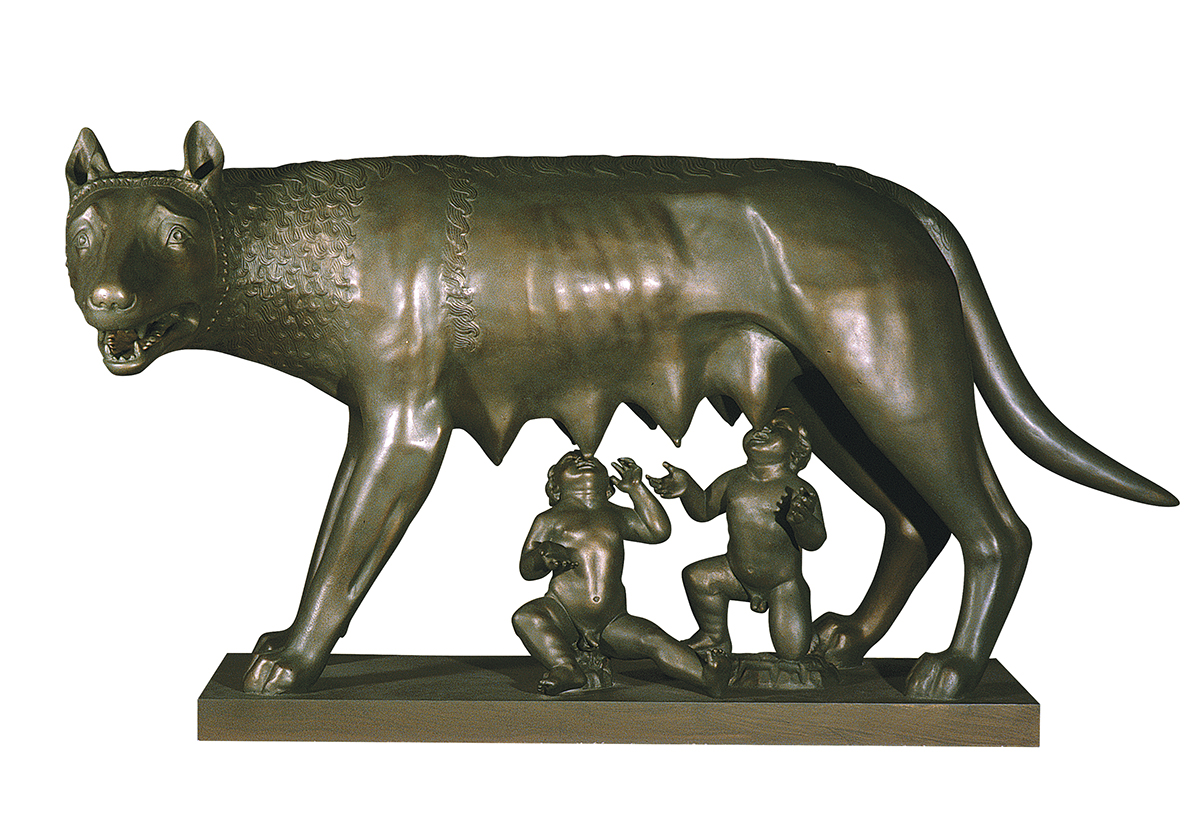The image shows a detailed bronze statue of a mythical animal that appears to be a mix of various creatures, resembling parts of a bear, cat, and dog. The animal, which has a distinctly open mouth with sharp teeth and expressive, slanted eyebrows, is captured in a seated position on a thick, bronze rectangular base. It has fur texture around its neck and a smooth body with visible ribcage definition. The statue has teats on its underside, from which two naked cherubic figures, evidently male, are drinking milk. The animal's head is turned towards the viewer, showcasing short hair and detailed features, while its body is oriented to the left side of the frame. The overall coloration of the statue is a blend of brown and gray tones.